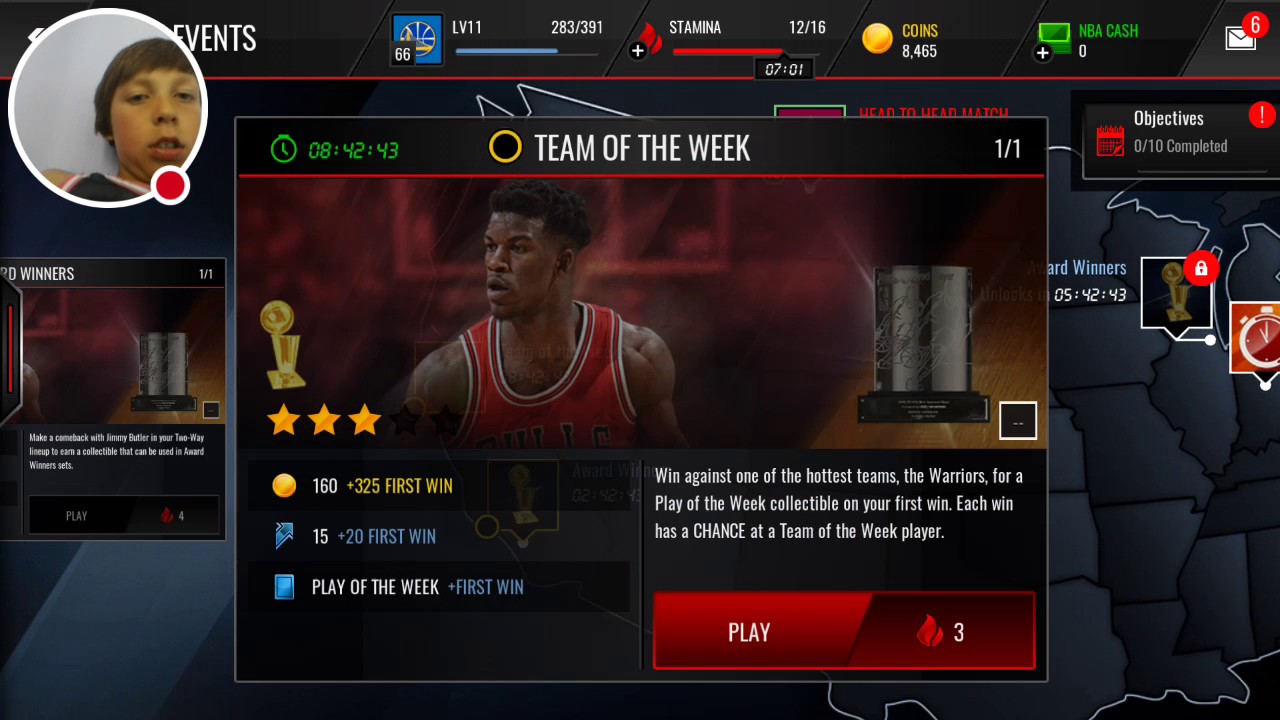This is a detailed screenshot of a sports-themed gaming website. In the top left corner is a profile icon of a young man, accompanied by a red circle beneath his picture. The top section of the screen displays various player statistics: the user is on level 1 and has a progress bar showing 283/391, with stamina at 12/16, coins totaling 8,465, and an unspecified amount of NBA cash. An envelope icon in the top right corner indicates that there are 6 unread messages.

Dominating the center of the screen is a large banner titled "Team of the Week," with a countdown timer below it displaying 8 hours, 42 minutes, and 43 seconds. Next to this banner, it shows a 1/1 indicator and features an image of a basketball player alongside a trophy with 3 stars. The panel below provides various stats: "160/325" and "First Win: 15/20," indicating some progress or achievements. 

The image advertises a challenge to win against the popular team, the Warriors, with the reward being a play-of-the-week collectible on the first win. It further mentions that each victory offers a chance to earn a team-of-the-week player. The background of the site is dark, resembling a map, but some icons are partially visible and unidentifiable.

At the bottom of the screen, a prominent red box displays the word "Play" along with an associated icon and the number 3.